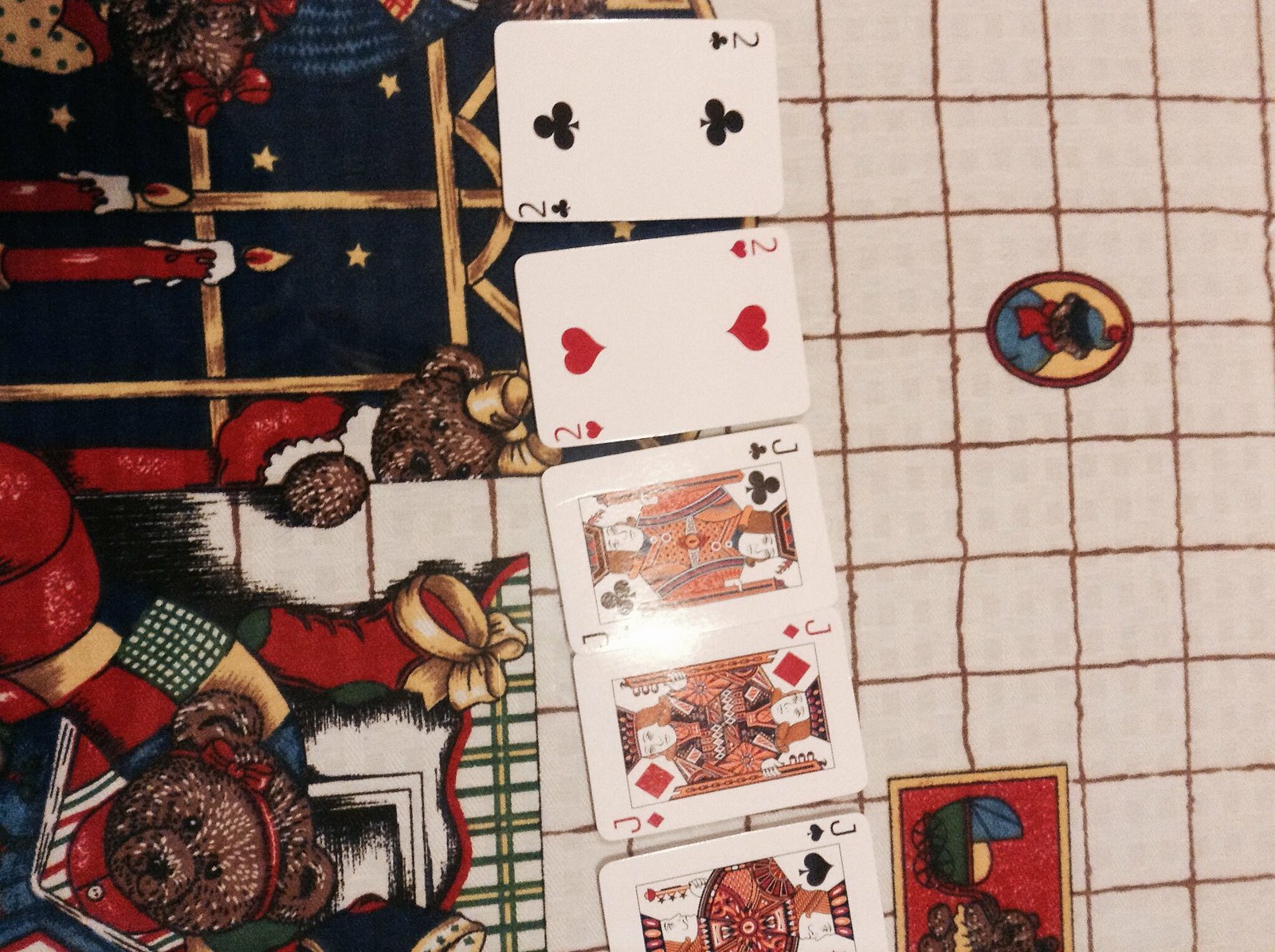This landscape-style image showcases various elements seamlessly integrated into a cozy scene. On the left side, a rug features an intricate design with two bears; one bear is half-visible, peeking through a door, while the other sits in front of a glowing fireplace adorned with two stockings hanging above it. The bears are oriented such that you need to tilt your head to the right to see them properly.

Centrally positioned in the image are five playing cards, arranged in a horizontal fashion but aligned vertically in a row. The hand includes a two of clubs, two of hearts, jack of clubs, jack of diamonds, and jack of spades.

On the right side, a plaid-patterned background catches the eye with its light brown hue and white grid lines, creating a graph-like appearance. This background texture resembles a rug or carpet, complete with an oval-shaped medallion in the center, depicting a small, rotated bear, adding to the overall whimsical and warm atmosphere of the image.